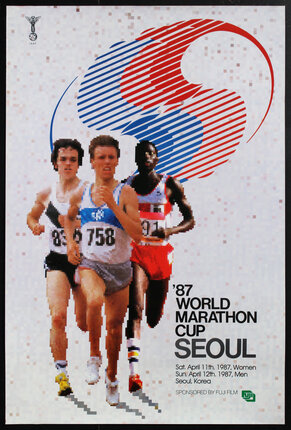This is a vibrant poster advertising the 1987 World Marathon Cup in Seoul, South Korea. The event took place on Saturday, April 11th, 1987 for women, and Sunday, April 12th, 1987 for men, and it was sponsored by Fujifilm. The top half of the poster is dominated by an oval-shaped logo featuring horizontal lines forming an 'S' shape, colored blue on the left and red on the right, with a yin-yang-like shape next to the 'S'. 

In the bottom left third of the poster, three male runners are depicted in mid-stride, running towards the camera. The central figure is a light-skinned man wearing a white tank top with a blue stripe and the number 758, paired with gray shorts. To his left is another light-skinned man in a white tank top with a black stripe and black shorts, wearing the number 83. On the right, a dark-skinned man wears a white tank top with an orange stripe and orange shorts, marked with the number 91. 

The poster is rich in blue and red, which may reflect the colors of the Korean flag, and gives a dynamic and colorful impression of the event. The text detailing the event, "87 World Marathon Cup Seoul, Saturday, April 11th, 1987, women, Sunday, April 12th, 1987, men, Seoul, Korea, sponsored by Fujifilm," appears in black on a gray background in the bottom right corner. Adjacent to this text is the green Fuji logo. Additionally, in the top left-hand corner sits an icon resembling an angel with wings standing on a sphere, adding a unique touch to the overall composition.